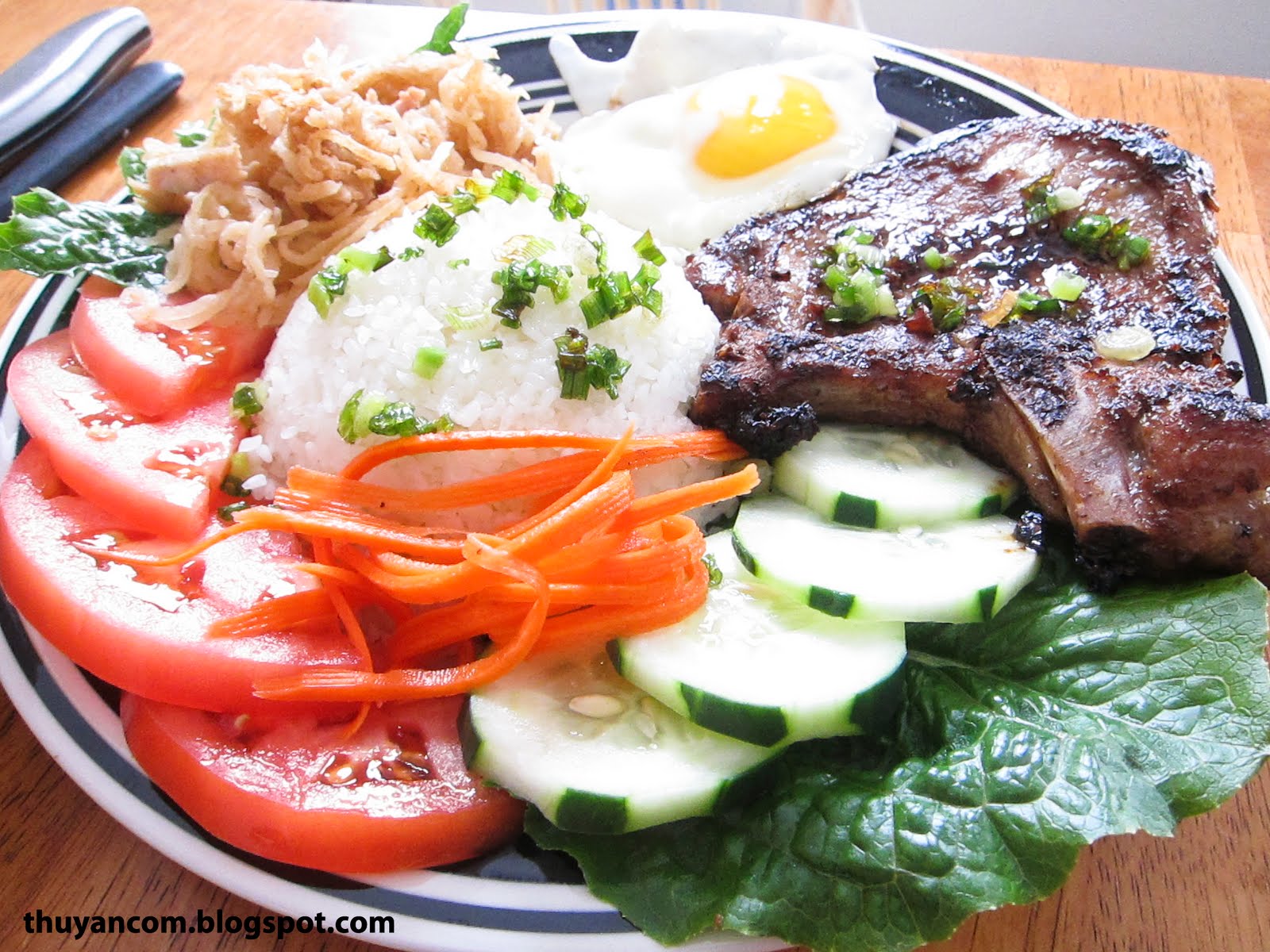This photo, originally posted on thancom.blogspot.com (as indicated by the watermark in the lower left corner), features an artfully plated meal, likely from a restaurant. The dish is presented on a large, white plate adorned with blue stripes along the rim. Centered on the plate is a generous portion of rice, garnished with a sprinkling of green herbs. To the right, a succulent piece of steak is accompanied by sliced cucumbers resting on a large green leaf. Above the rice, a perfectly fried egg commands attention. The left side of the plate showcases a serving of cooked ramen noodles, also laid on a green leaf, completing the intricate presentation. Below the rice, thin strips of shredded carrot and neatly arranged tomato wedges add vibrant color to the composition. The setting includes a wooden placemat on a sleek black tabletop, with utensils placed to the left of the plate. Soft reflections of light filter through a nearby window, casting a gentle glow on the tantalizing meal.